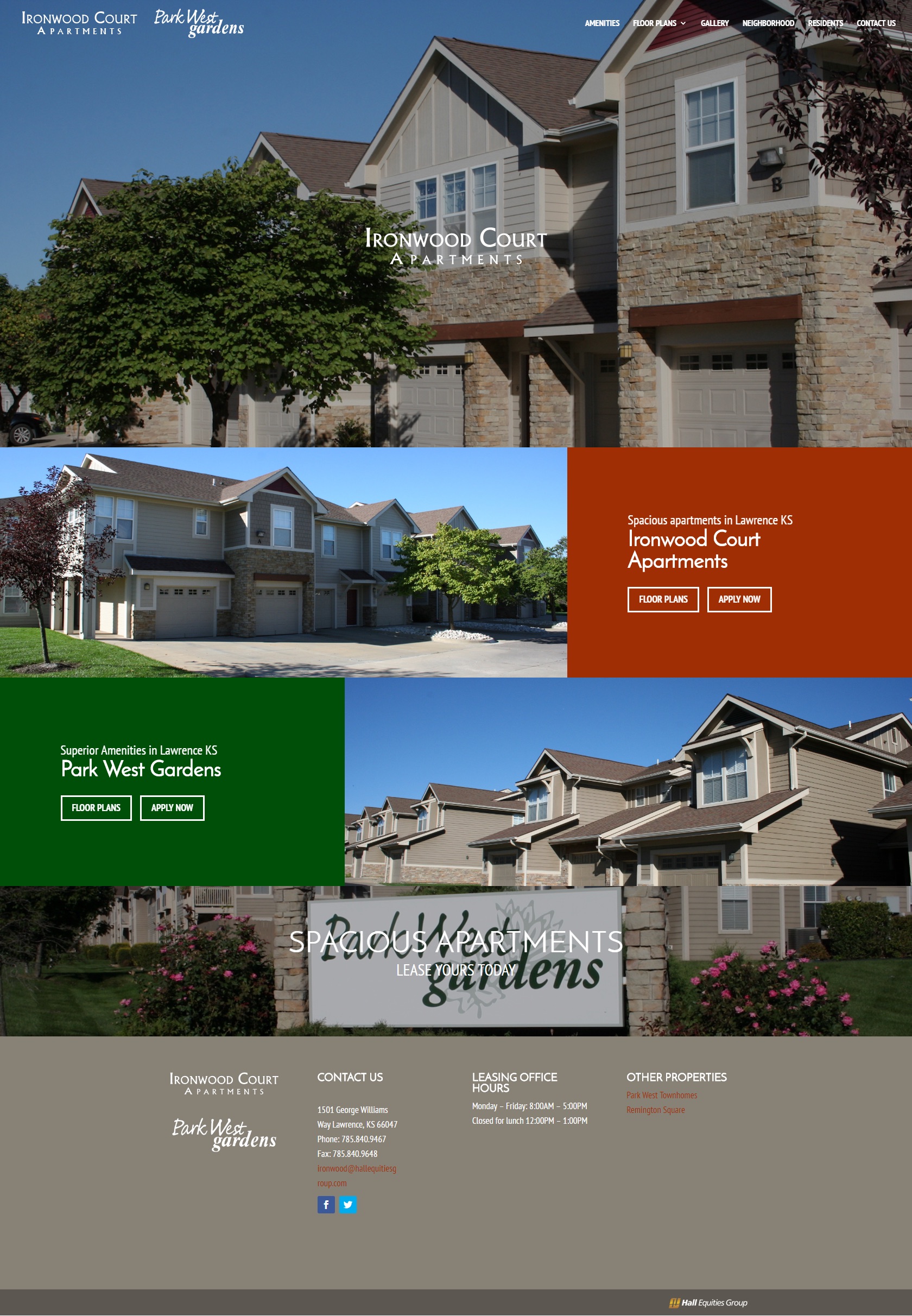A web page for a real estate listing is displayed, showcasing the Ironwood Court Apartments located in Park West Gardens, Lawrence, Kansas. The main image features a grey house with brown roofs, white garage doors, surrounded by dark green trees, and set against a dark blue sky. The visual provides various angles of the housing property.

At the top of the page, "Ironwood Court Apartments" is prominently highlighted in bold white font, with "Park West Gardens" elegantly written below in cursive bold white. On the right-hand side, there are navigation tabs also in bold white font, including options such as Amenities, Floor Plans, Gallery, Neighborhood, Residents, and Contact Us.

Centrally positioned, the name "Ironwood Court Apartments" is reiterated, this time accompanied by a smaller left-hand side image of the property. Within a distinctive red rectangle, it announces "Spacious Apartments in Lawrence, KS."

Further down, there are two interactive buttons: one with a white border labeled "Floor Plans" and another labeled "Apply Now." The apartment complex is illustrated again, facing right, highlighting the Park West Gardens sign, which includes two brick pillars and a white rectangle with black text reading "Park West Apartments," seemingly painted on.

In the upper left section of the sky, the text "Superior Amenities in Lawrence, Kansas, Park West Apartments" is depicted. The same two buttons, "Floor Plans" and "Apply Now," are repeated for user convenience.